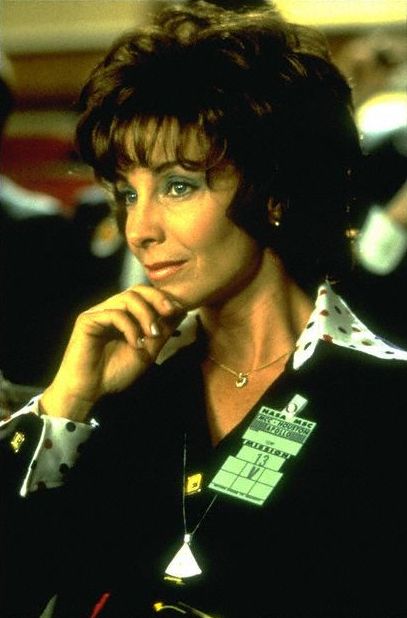This color movie still from "Apollo 13" features actress Kathleen Quinlan. She is seated and gazing thoughtfully to the left, with her chin lightly resting on her right hand. She is dressed in typical late 1960s fashion, with a black top and a white collared shirt beneath, both adorned with dark polka dots. Her wide-lapel jacket and large cuffs complement her ensemble, which is typical of the era. She has short, dark, shaggy hair with wavy bangs framing her face. Kathleen is wearing a small gold necklace that catches the light, adding a bright focal point towards the lower part of the image. She also sports matching gold earrings. Clipped to her blouse on the left side is an identification badge that reads "NASA MSC Houston Apollo 13," distinctly marked with the number 13 and a "V." The background, slightly out of focus, features a mix of red, black, white, and beige hues.